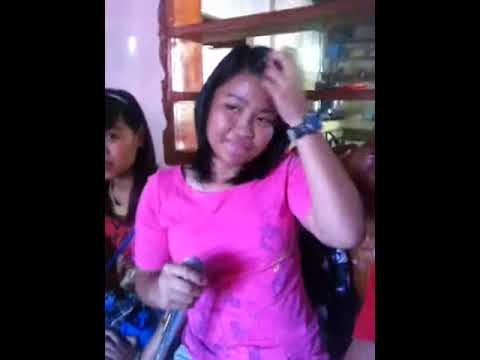In this color photograph, a young girl, resembling Filipino descent with darker skin and long black hair, is the central focus. She's wearing a pink shirt and holding a silver microphone with a black cord in front of her mouth, using both hands to grip it near the top. Her eyes are directed towards the top right corner, suggesting she might be reading lyrics off a monitor, indicating she could be singing or giving a speech. A black wristwatch adorns her wrist. To her left, another girl with a similar darker complexion and black hair styled in a ponytail is visible, though only the side of her head is seen as she looks out of frame to the left. The setting appears to be indoors, possibly at a karaoke or party event, given the casual yet engaged posture of the subjects. The background features a pale pink wall and a wooden cabinet or shelving unit behind the central figure, adding a domestic or informal ambiance. The photograph, taken in portrait orientation, is inset into a landscape background of black, emphasizing the focused and representational realism of the scene. The image shows no text, with colors prominently featuring off-white, black, brown, blue, pink, purple, tan, and red.